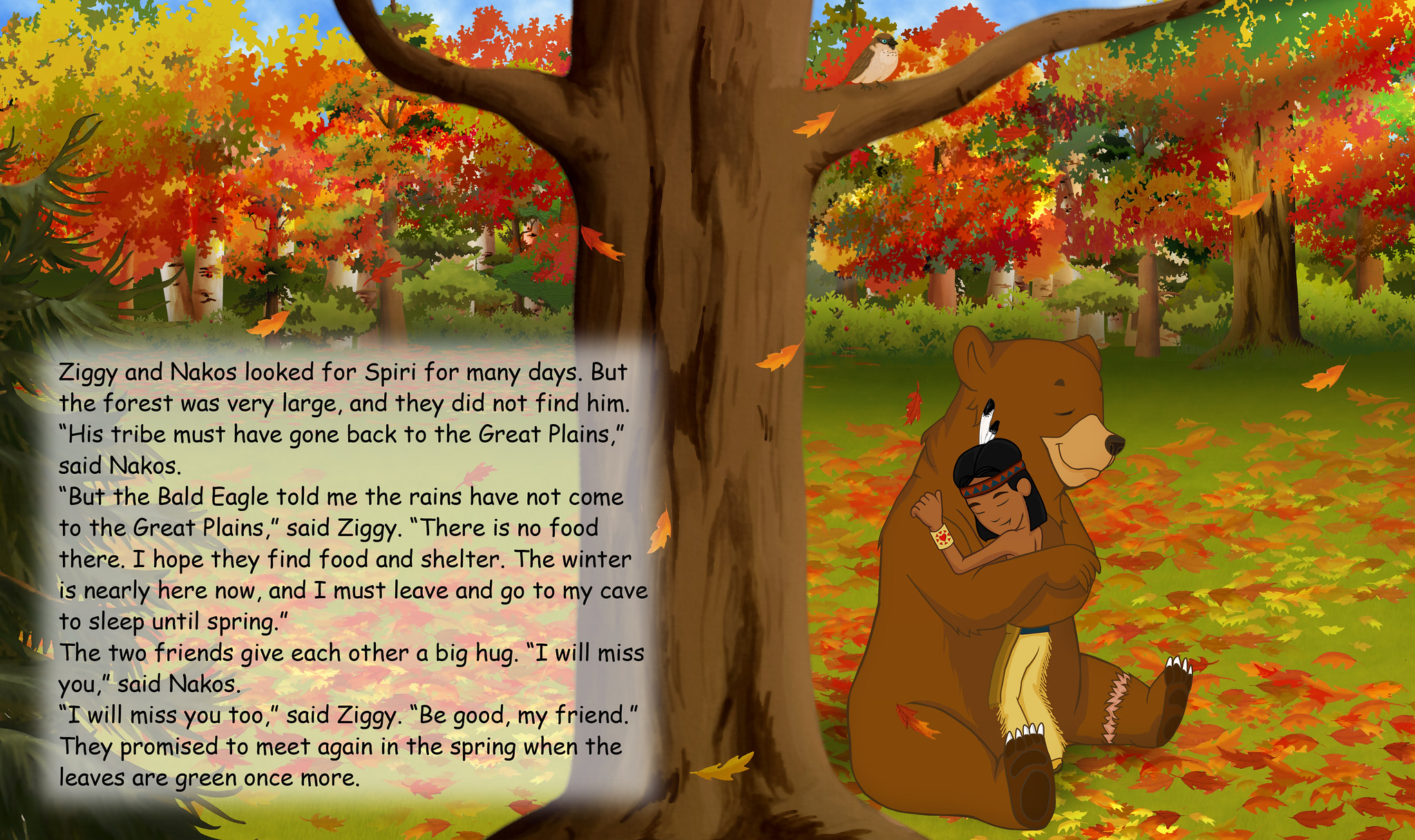This rectangular illustration, roughly six inches wide and three inches tall, appears to be taken from a children's book. Dominating the center is a cartoon drawing of a tree trunk, surrounded by trees adorned with red, yellow, orange, and green leaves, with some leaves gently falling, indicating the autumn season. To the right of the tree, a large brown bear with a wound on its leg sits on the ground, hugging a smiling Native American boy, who wears a feather and headband. Both the bear and the boy are smiling. There's a small bird perched on a limb above them. To the left of the tree is a semi-transparent white box with faded edges containing black printed text. The text narrates the story: "Ziggy and Knackos looked for Spearie for many days, but the forest was very large and they did not find him. 'His tribe must have gone back to the Great Plains,' said Knackos. 'But the bald eagle told me the rains have not come to the Great Plains,' said Ziggy. 'There is no food there. I hope they find food and shelter. The winter is nearly here now and I must leave and go to my cave to sleep until spring.' The two friends gave each other a big hug. 'I will miss you,' said Knackos. 'I will miss you too,' said Ziggy. 'Be good, my friend.' They promised to meet again in the spring when the leaves are green once more."